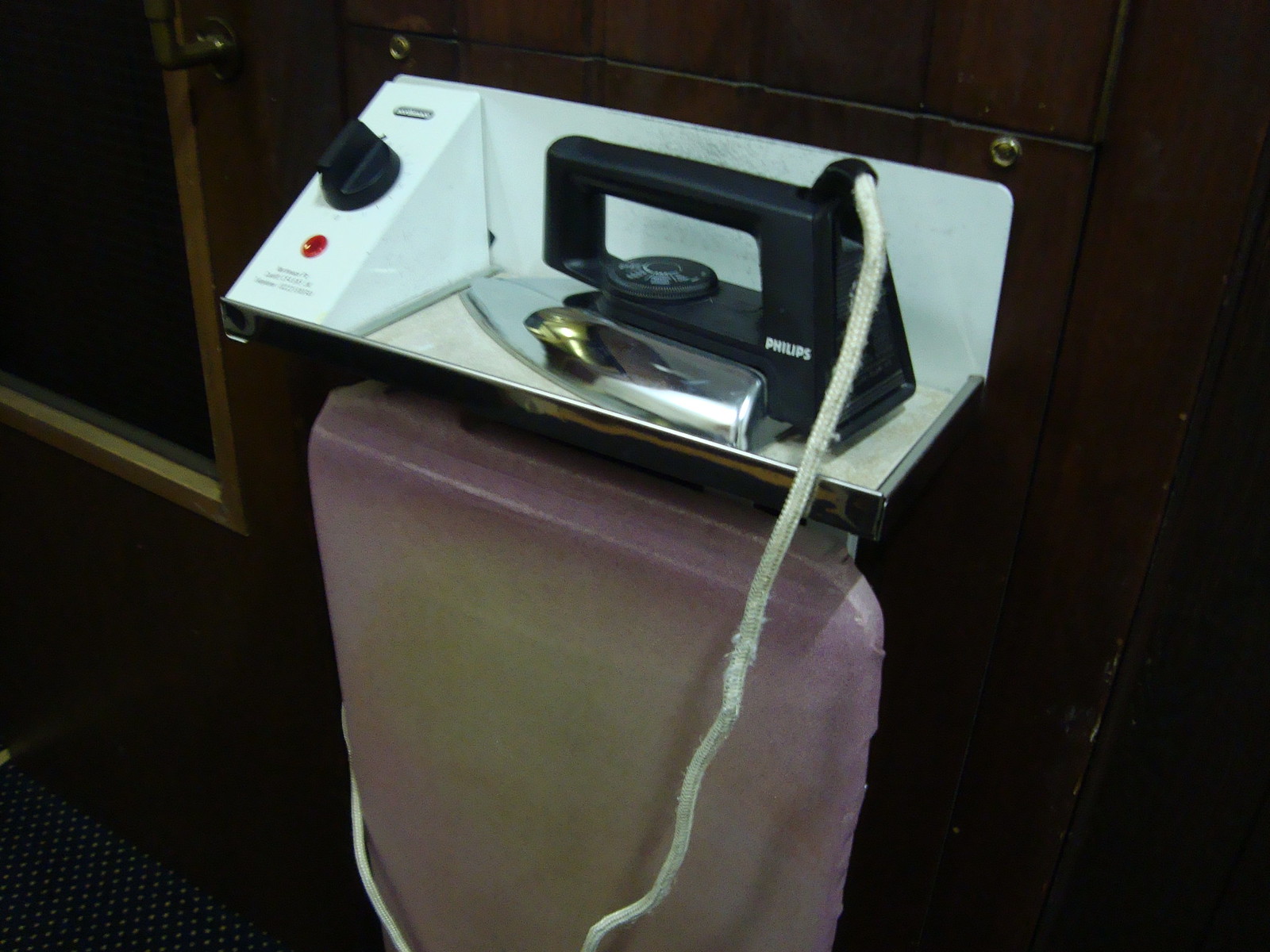This photograph shows an antique-style Philips iron with a black plastic handle and a stainless steel bottom. The iron is fitted with a frayed white cord that extends from the handle, trailing off towards the floor. Prominently displayed on the black handle is the Philips logo in white. The iron is equipped with a small control knob, presumably for adjusting the heat level. It rests on a white receptacle, possibly designed to hold water, which also features a black knob, a red indicator light, and some white metal components. The entire setup appears to be mounted on a wooden wall with a door on the left side. The presentation suggests a museum display, providing an insightful glance into the history of household appliances.